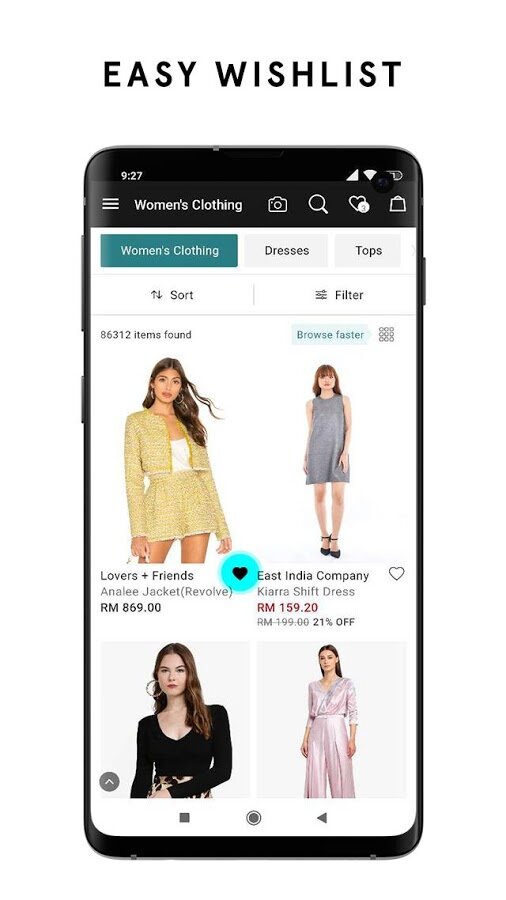This image showcases a black cell phone under the heading "Easy Wishlist," which appears on its screen. The photograph is not a screenshot but an actual picture of the cell phone, revealing all its edges including visible buttons. The phone is oriented backwards, showing login buttons on the left, a power button below them, and an additional button on the top right. In the top left corner of the screen, the time "9:27" is displayed in bold white text, accompanied by a full set of carrier bars and another icon that resembles a full black eye. There is an unrecognized symbol on the far right.

The interface under the hamburger menu reads "Women's Clothing." Various icons are present, including a camera, a magnifying glass, a heart with a white circle at the bottom featuring a possibly unreadable number, and what looks like a clipboard. The main part of the screen is white. In the upper left corner, inside a green box, it says "Women's Clothing" in white text, alongside additional categories like "Black Dresses" and "Blackboard Tops" in white boxes. Below a gray dividing line, options for sorting and filtering items are displayed. The screen reports "86,312 items found" in black text and encourages users to "Browse Faster" in green text within a light green box.

Prominently featured are images of women modeling clothing. One woman wears a yellow miniskirt and matching short jacket over a white tank top. She has long brown hair, dangly earrings, red lipstick, and brown eyes, posing with a hip cocked out holding a bag in her right hand. Below her image, text reads "Lovers and Friends Annalie Jacket (Revolve)", priced at RM869, with a teal circle around a black heart.

Adjacent is another model in a gray sleeveless dress that ends mid-thigh, wearing ankle-strap sandals. The text beneath her image states "East India Company Kiara Shift Dress" priced at RM159.20, with an original price of RM199.00 crossed out indicating a 21% discount.

Towards the bottom left, another woman with brown hair wears a tight-fitting V-neck long-sleeved black shirt paired with a cheetah belt, and a cheetah print skirt is visible. On the right, a model in a light pink silky outfit, both pants and a V-neck shirt, stands with her hands at her sides. Navigation icons below include a square, circle, and left-hand arrow, suggesting that the displayed device is a Samsung phone.